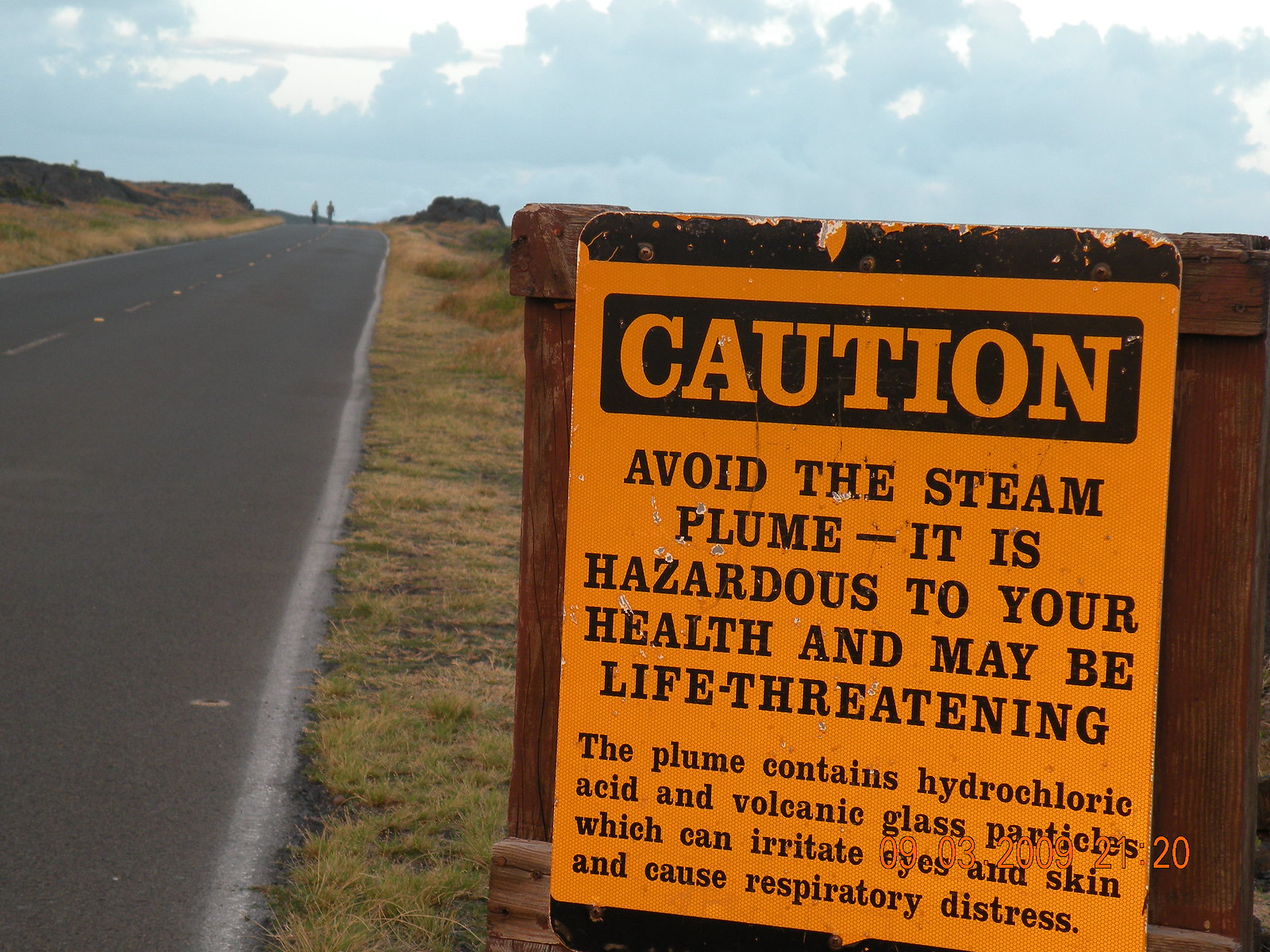This wide, rectangular image features a cautionary sign next to a road that extends from the bottom left corner into the horizon just below the top left corner. The dark gray road, with its dotted yellow center line and grayed white edge lines, is bordered by brownish green grass extending up a hill. The sign, made of yellow metal with a black border at the top and bottom, is mounted on a dark brown, square-shaped wooden post located on the right side of the image. The sign's message, highlighted in black with orange text, reads: "Caution." Below, in black text, it warns, "Avoid the steam plume. It is hazardous to your health and may be life-threatening. The plume contains hydrochloric acid and volcanic glass particles, which can irritate eyes and skin and cause respiratory distress." In the distant horizon, two people are visible standing in the middle of the road under a predominantly white sky with light blue clouds.